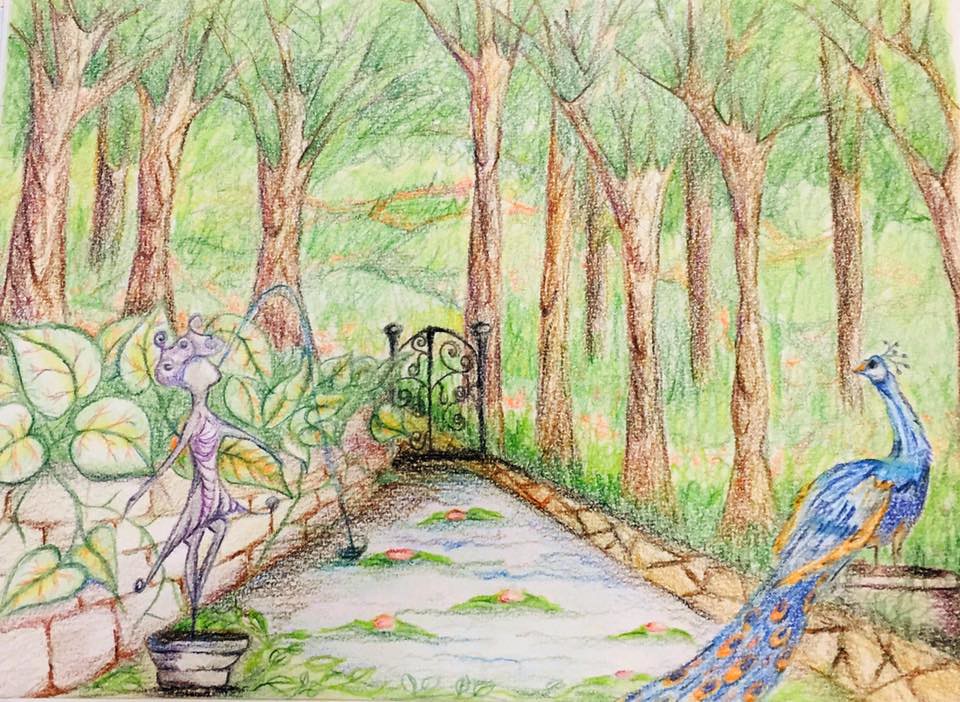This image is a photograph or scan of a color pencil drawing executed on heavily textured paper, giving it the appearance of canvas. The drawing portrays an outdoor landscape scene dominated by leafless trees occupying the upper two-thirds of the composition. Below the trees, a lush green field stretches out, grounding the scenery and providing a serene backdrop.

In the foreground, a stone path extends from the viewer's perspective, drawing the eye straight towards an intricately detailed wrought-iron gate rendered in black pencil. The gate stands as a focal point, enhancing the depth and inviting the viewer into the landscape.

On the lower left side of the drawing, a potted plant houses a fairy sculpture, adding a whimsical touch to the natural setting. On the opposite lower right side, a beautifully illustrated peacock perches gracefully on a small section of the fence along the path, its vibrant plumage contrasting with the muted tones of the trees and the gate. The scene meticulously combines elements of fantasy and natural beauty, creating a captivating and detailed visual narrative.